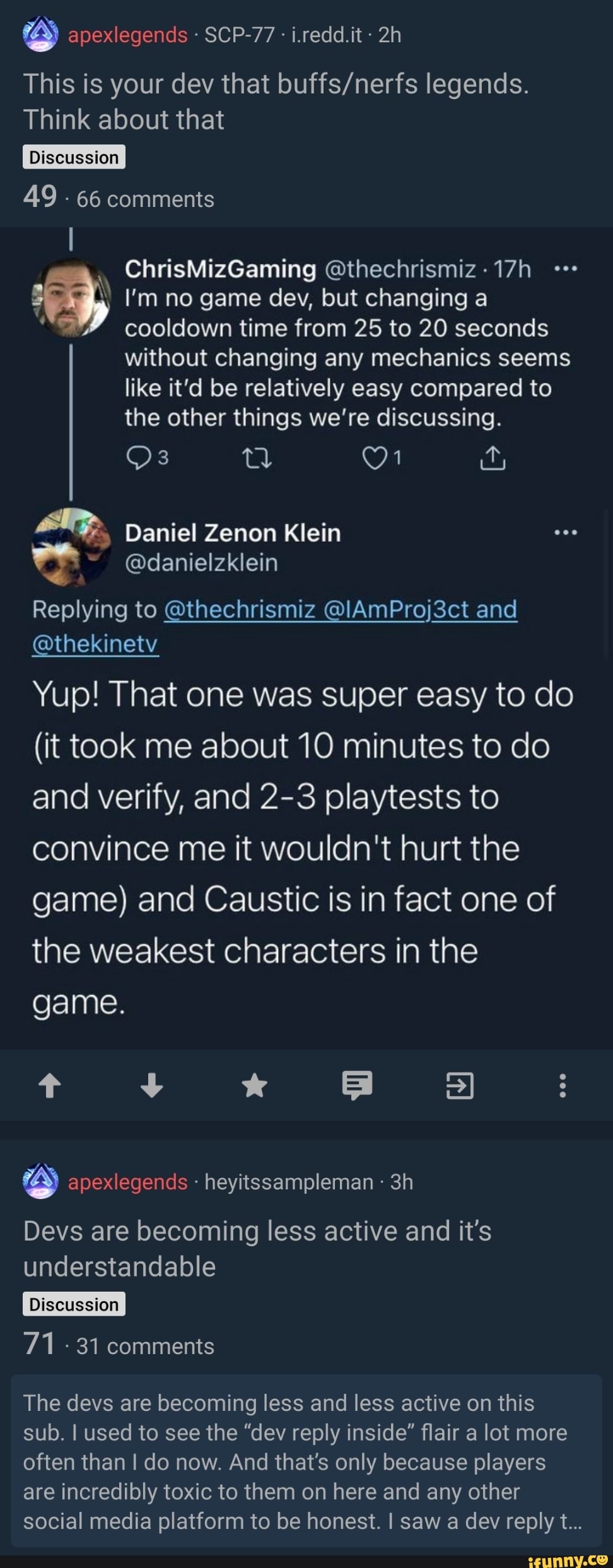This image showcases a series of Twitter posts discussing the development and community interactions surrounding Apex Legends. At the top, a user mentions, "Us, Apex Legends," followed by a statement: "This is your dev that buffs, nerfs, slash nerfs legends. Think about that."

The conversation continues with Christmas Gaming responding, "I'm no game dev, but changing a cooldown time from 25 to 20 seconds without changing any mechanics seems like it'll be relatively easy compared to the other things we've been discussing."

Daniel Zenon Claim then chimes in, agreeing: "Yep, that one was super easy to do. It took me about 10 minutes to do and verify and 2 to 3 play tests to convince me that it wouldn't hurt the game."

The next part of the discussion highlights that "Encaustic is in fact one of the weakest characters in the game."

At the bottom of the image, another post raises a concern about developer participation: "By Apex Legends, devs are becoming less active and it's understandable. The devs are becoming less active and less active. Less and less active on this sub. I used to see the dev reply inside. Flare Flare a lot more often than I do now and that's only because players are incredibly toxic to them on here and any other social media platform to be honest."